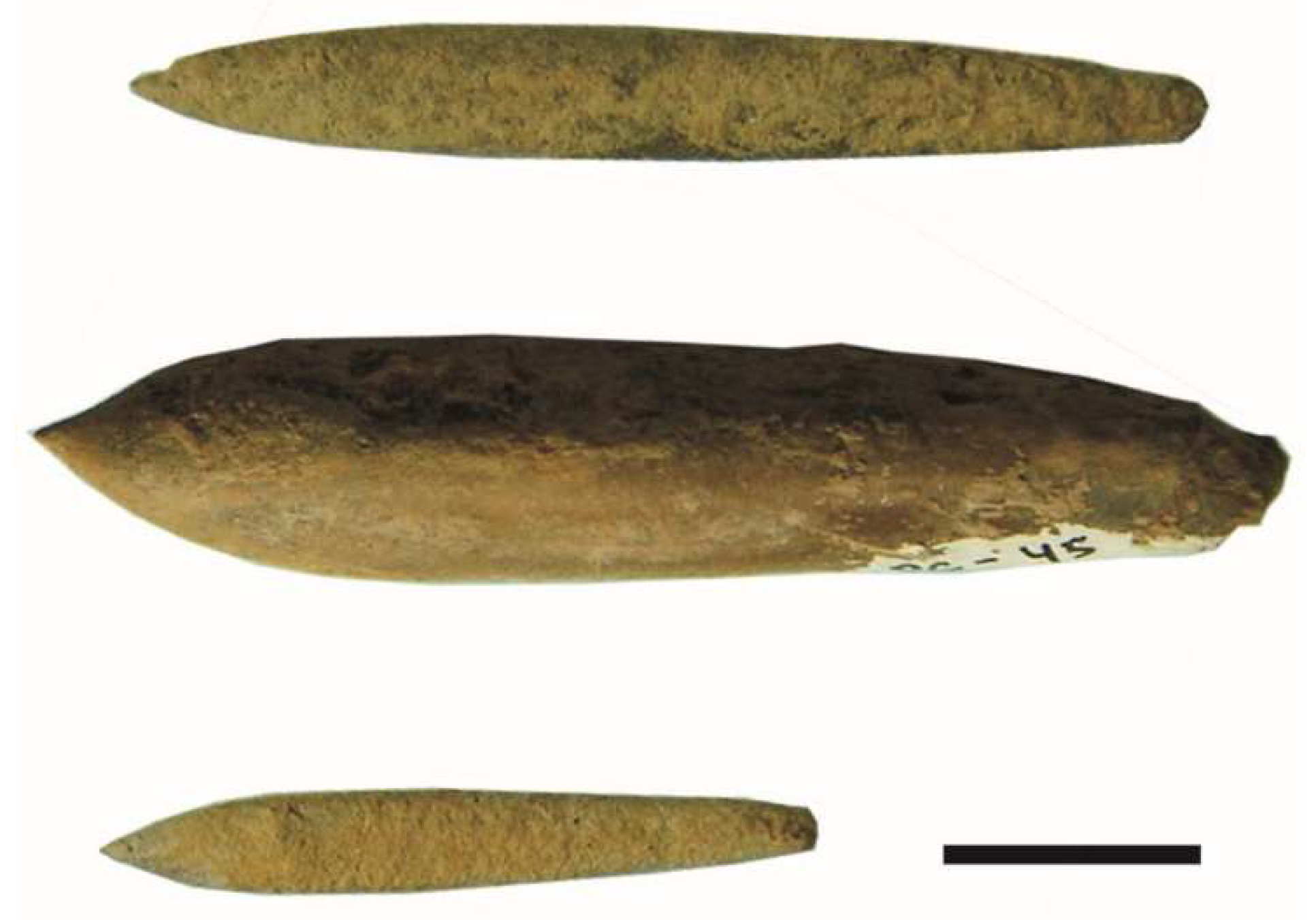The image displays three tubular, cigar-shaped rocks of varying sizes, arranged horizontally against a white background. The top rock, medium in size, is brown with dark brown or black flecks, featuring a pointed end on the left and a rounded end on the right. It is slightly thicker in the middle. The centrally positioned rock is the largest, running from top to bottom with a shadow on its top portion that gives it a darker appearance. It has a pointed tip on the left and a black marking near its bottom right that includes the number "45." The smallest rock is at the bottom, also cigar-shaped with a pointed left end and a blunt right end, and sits beside a solid black bar. All three rocks have a textured surface, enhancing their natural appearance.